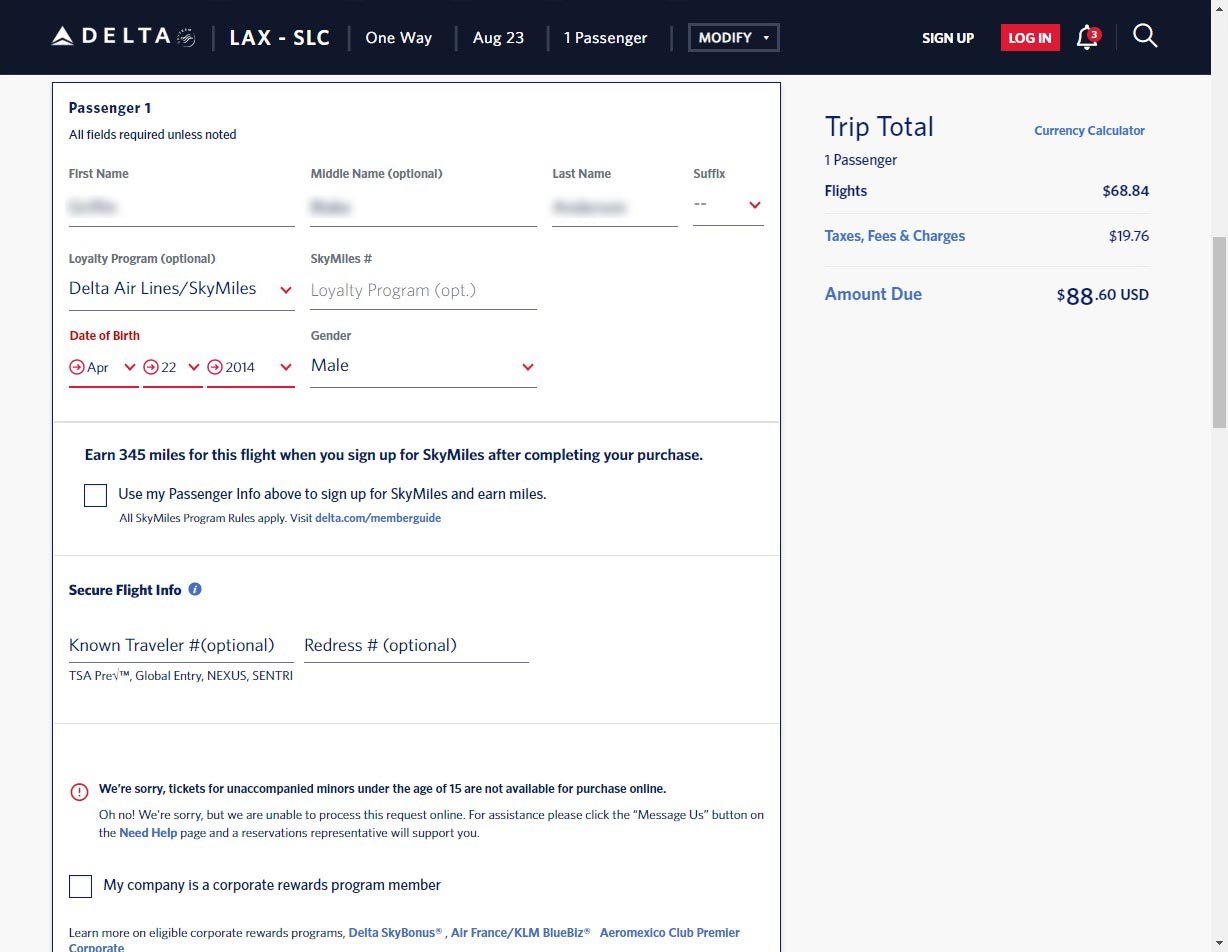Caption: 

The top section of the booking webpage displays details for a one-way Delta flight from Los Angeles (LAX) to Salt Lake City (SLC) on August 23rd for one passenger. To the right of these details, there are options to modify the search, a prompt to sign up, and a red login button. A notification bell with a red alert icon and a magnifying glass for search functionality are also present. 

On the right side, the trip summary indicates a total amount due of $88.60 USD for one passenger. This includes $68.84 for the flight itself and an additional $19.76 for taxes, fees, and charges. Below this summary, a link to a currency calculator is available.

On the left side of a large input box, titled "Passenger One," users are prompted to fill in all required fields unless otherwise noted. The fields include sections for the first name, middle name, last name, and suffix, which are blurred out in the image. There's also an optional field for a loyalty program, specifically Delta Airlines SkyMiles.